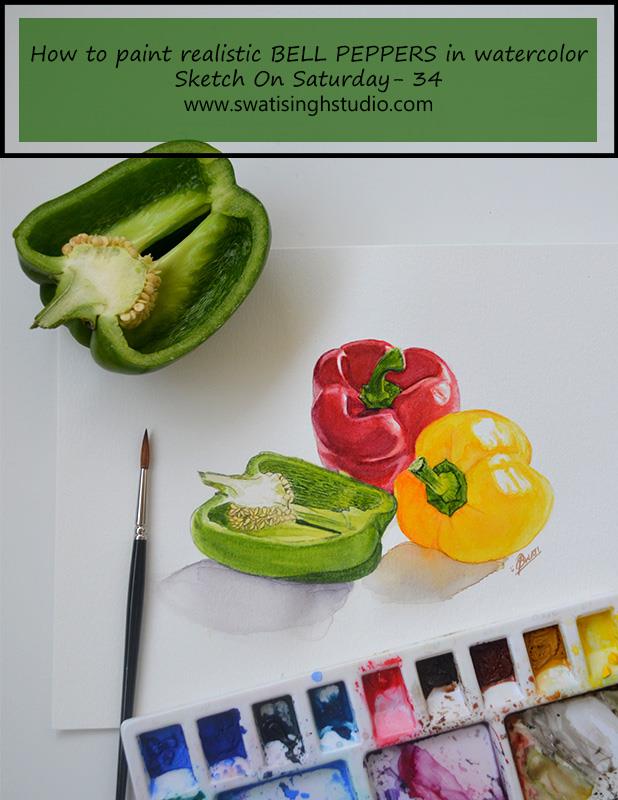The image is an advertisement for an art class titled "How to Paint Realistic Bell Peppers in Watercolor." The top section features a green rectangle with a white border and black outline, containing the text: "Sketch on Saturday, 3-4," and "wswatsinghstudio.com." Below this, on a white surface, sits a real green bell pepper cut open on a piece of white drawing paper. Surrounding the real pepper are watercolor paintings of three bell peppers: one red, one yellow, and a similarly cut open green pepper. A paintbrush rests on the paper, accompanied by a white carton holding various watercolor paints in different stages of use, alongside a larger mixing palette.